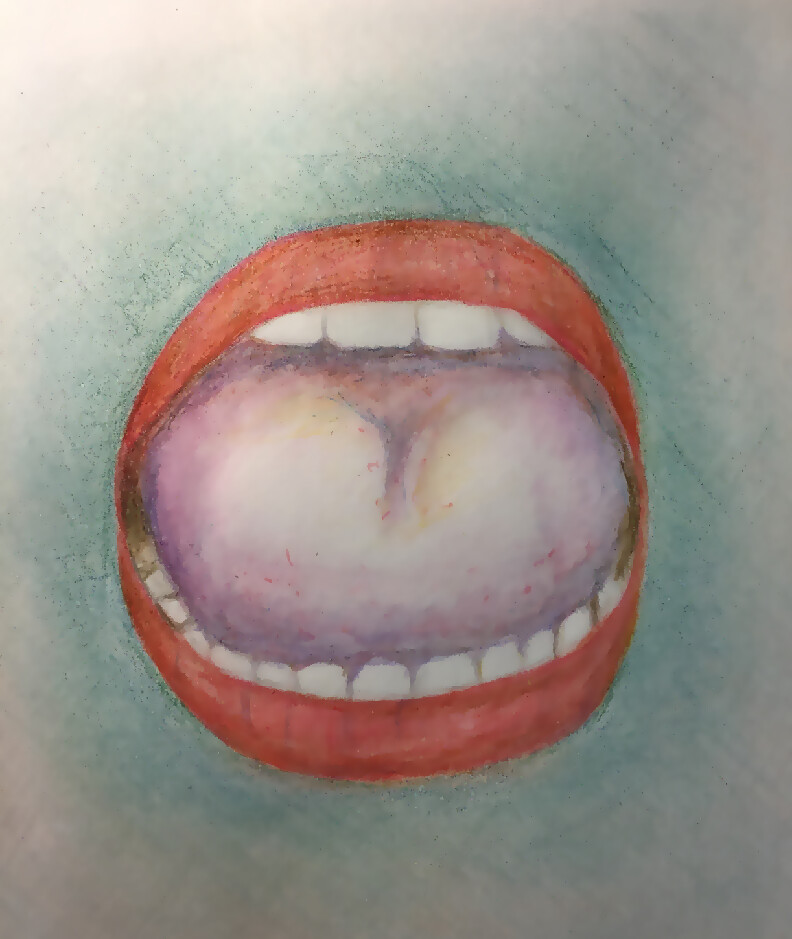This detailed colored charcoal sketch portrays an open mouth in striking detail. The central focus is the mouth, with vibrant red lips framing the scene. The tongue, prominently pink and appearing swollen, occupies much of the mouth's interior. The teeth, pearly white, are visible on both the top and bottom jaws, with a slightly higher number on the bottom. Surrounding the mouth, the backdrop transitions from a greenish hue to a natural skin tone, suggesting the contours of a face. The use of colored charcoal gives the piece a textured, sketch-like quality, emphasizing the mouth's dynamic and expressive features.